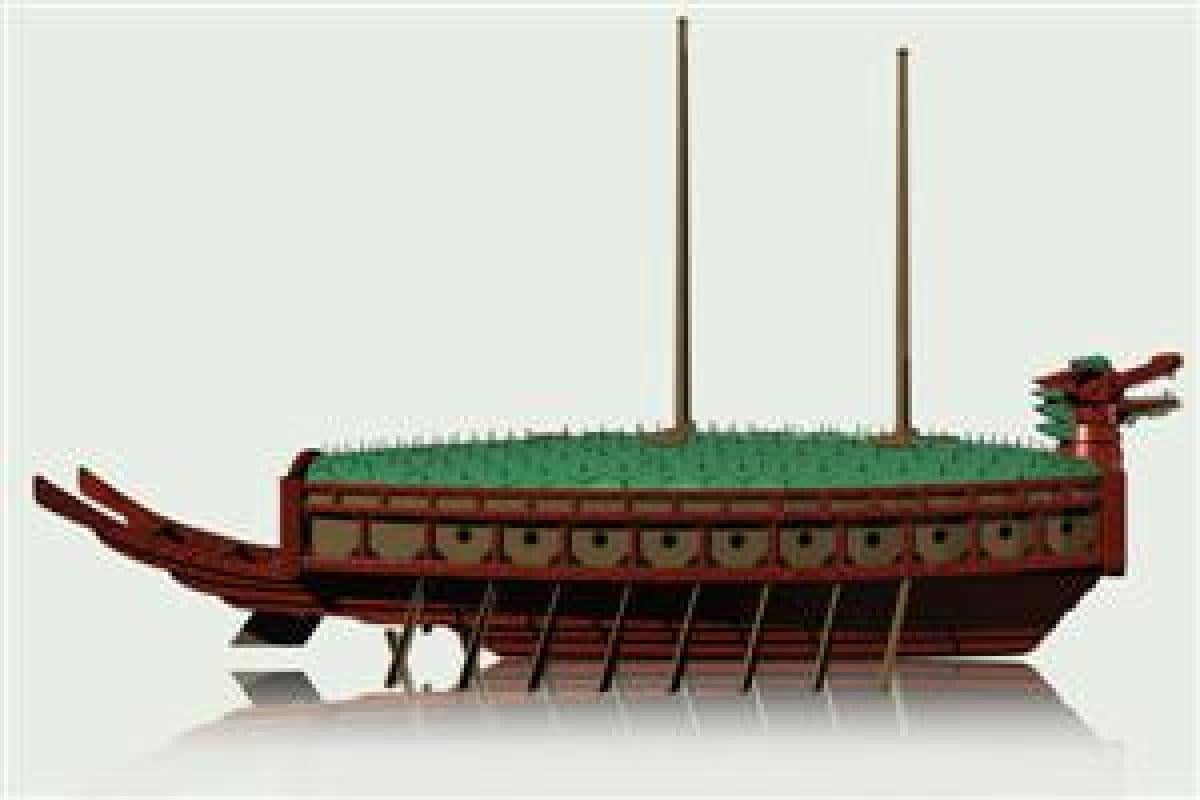This detailed image showcases a digitally-rendered model of an ancient boat, likely inspired by Viking or traditional Chinese designs. The backdrop is a mix of gray and white tones, with the boat’s central focus standing out prominently. The boat is characterized by its reddish-brown wooden hull, which houses eight paddles extending from its sides, indicating that it would have been rowed by numerous individuals below deck.

The deck itself is strikingly green, complimented by the vibrant red dragon figurehead at the prow, its mouth agape and eyes fierce. This dragon motif continues at the stern with twin dragon tails and a fin, emphasized in red, adding to the vessel's ornate design. Onboard, two vertical poles, akin to masts, rise upwards, suggesting the potential for sails, merging rowing with sailing capabilities.

Decorative black dots form a repeating pattern along the sides, enhancing the intricacy of the ship’s design. The image has a slightly blurred edge, reinforcing a digital or illustrative quality, and the boat rests on a subtly depicted surface. The model’s overall craftsmanship skillfully blends elements of historical shipbuilding with artistic embellishments, creating a vivid and detailed representation.